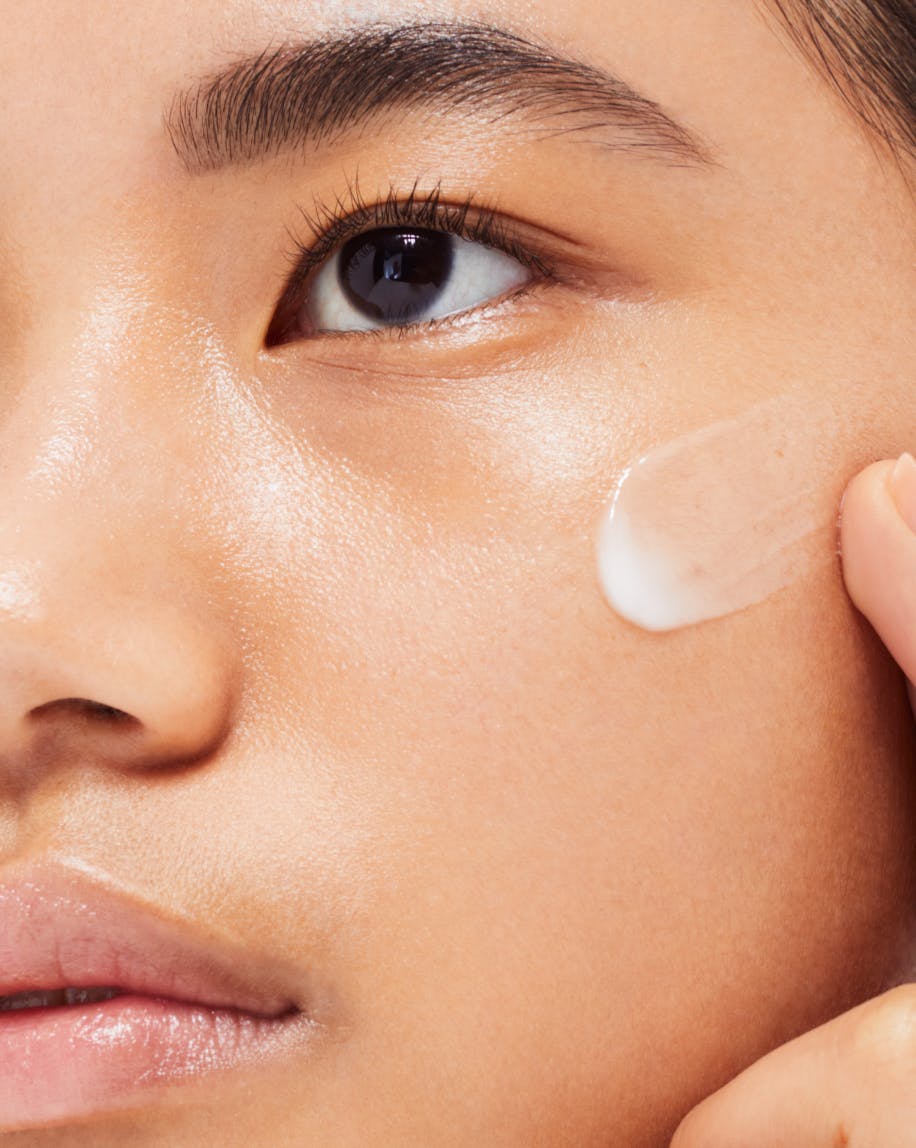This close-up, highly realistic photograph showcases the left side of a young Asian woman's face. Her smooth, dewy skin is a prominent feature, highlighted by a glossy pink sheen on her more-than-half visible lips, indicating the use of lip gloss. She has dark brown eyes and well-groomed brown eyebrows. Her gaze is slightly off-camera, with her face slightly turned to her right from our perspective, giving a clear view of her left eye and cheek. She is in the process of applying a streak of white moisturizer to her upper left cheekbone, just below and to the right of her eye, using one of her fingers. The moisturizer is spread horizontally across her cheek. Dark brown hair frames the rest of the visible face, enhancing the intimate and detailed nature of the close-up.